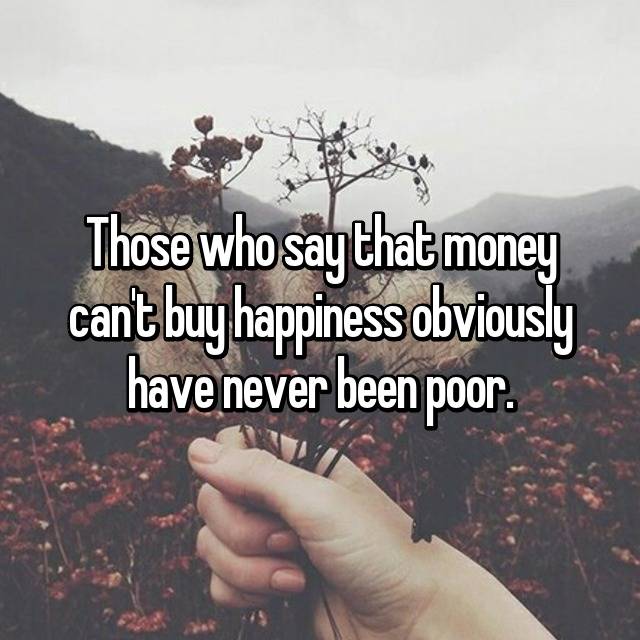The image is an inspirational meme featuring a poignant quote in white text with black borders that reads, "Those who say that money can't buy happiness obviously have never been poor." The text is superimposed over a photograph of a gray, overcast day. In the foreground, a person's right hand is holding a sad-looking bouquet of dead or dried-out flowers. The arrangement includes stems with no petals, dried blossoms, and a cotton ball-like plant. Some of the flowers have remnants of brown, withered petals, while others are just bare, dried stems with little stubs where flowers used to be. The background of the image features a foggy, wildflower-strewn field, with patches of reddish flowers hinting at life amidst the bleakness. Green hills and distant mountains rise in the backdrop, adding to the scene's somber, reflective atmosphere.